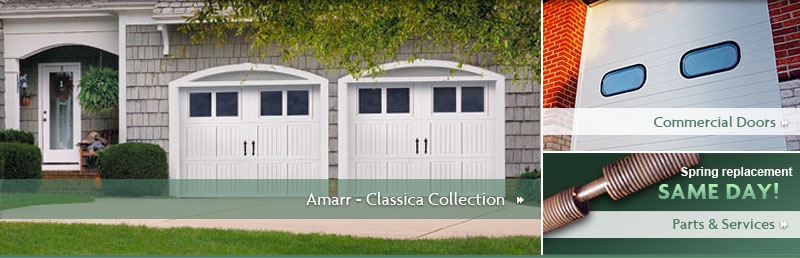The image consists of a website graphic laid out in three distinct panels. The left panel, which is the largest and rectangular in shape, features an outdoor setting of part of a house. This section prominently displays a gray facade with two side-by-side garage doors topped with arched windows. Surrounding the structure are lush trees and hedges. There’s also a white-framed entrance door to the house, accompanied by a chair with a figurine, a hanging basket, and a potted fern. At the bottom of this panel, a light green banner reads "Amarr Classica Collection" in capital letters, specifically spelled as "A-M-A-R-R - Classica."

The right panel is vertically divided into two sections. The top section showcases a red building with a visible garage door, overlaid with the text "Commercial Doors" in green on a white banner. The bottom section features a green background with an image of a spring and the text "Spring Replacement, Same Day" in green, with "Same Day" emphasized by an exclamation point. At the bottom of this section, a white banner carries the text "Parts and Services" in green.